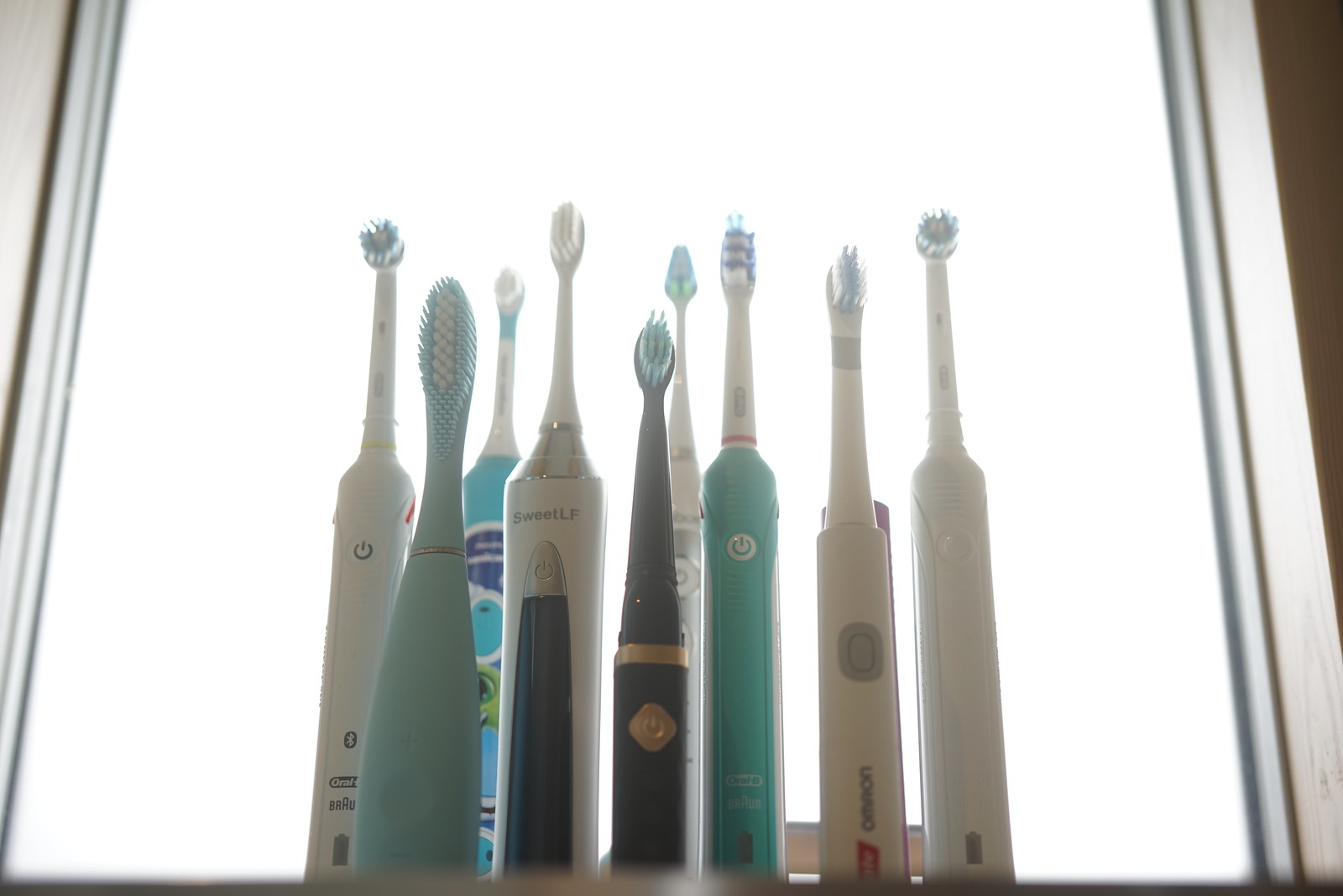The framed photograph showcases nine distinct styles of electric toothbrushes, precisely lined up in a row against a brightly lit white background. The toothbrushes, each differing in shape, size, and color, create a meticulously organized, military-like sentinel arrangement. Most have white or blue bases, with one sporting a black base. Among the varied toothbrush designs are round, oblong, oval, and even a uniquely teal one with a large, screwdriver-shaped bristle. Many appear rechargeable, though a brighter blue one in the back likely uses a D-size battery. Visible logos, such as those from Braun, and on/off buttons add further detail to the tableau of dental hygiene instruments.